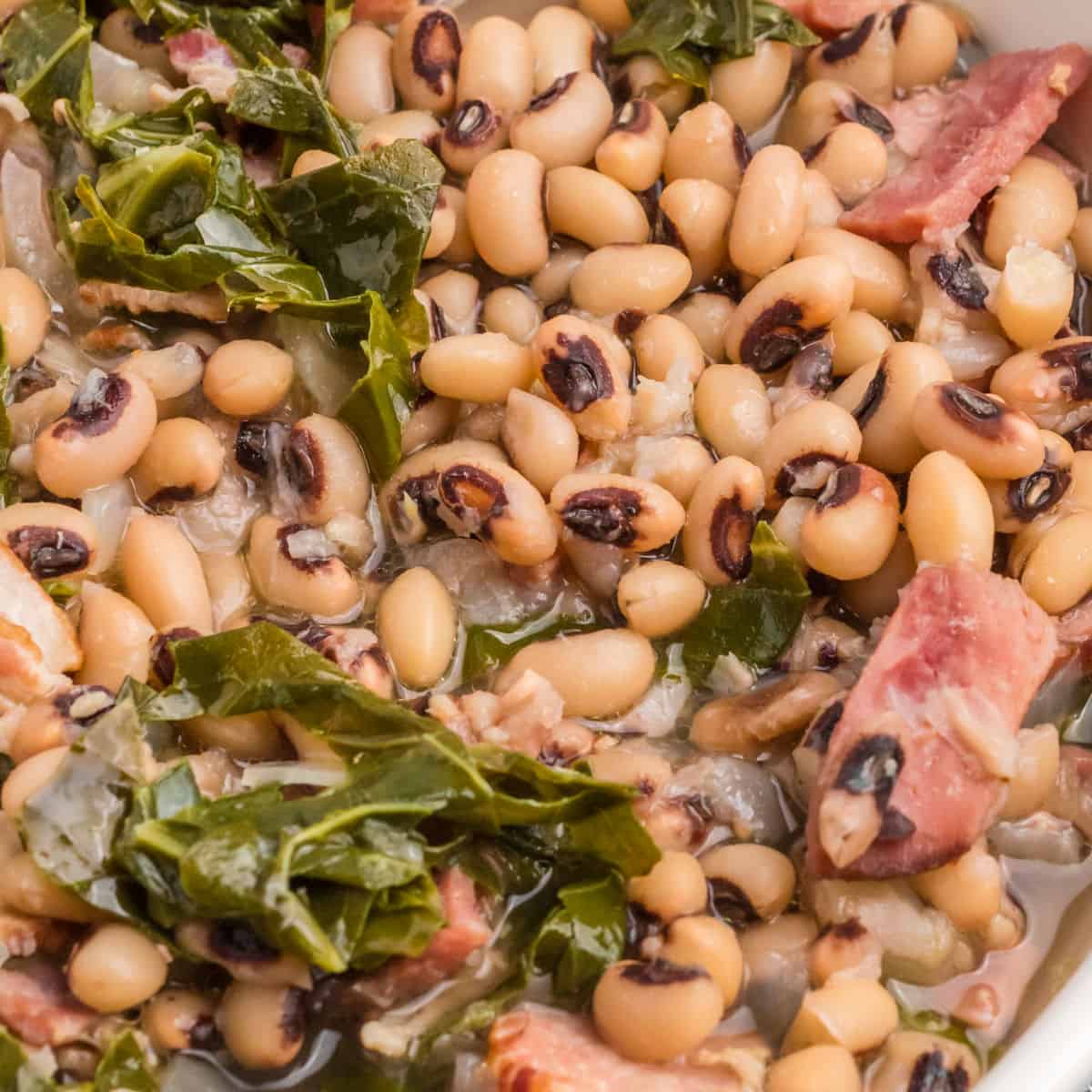This detailed photograph features a savory, cooked dish centered around beige black-eyed peas with characteristic dark brown centers. The meal also includes pieces of pink meat, varying from light to dark hues, which appear to be bacon. Mixed throughout the dish are shiny, dark green leafy pieces, likely spinach, along with some translucent white pieces that resemble onions. Everything is coated in a liquid, creating a cohesive and appetizing presentation, and the image captures the entirety of the dish, giving a close-up view of the various ingredients.